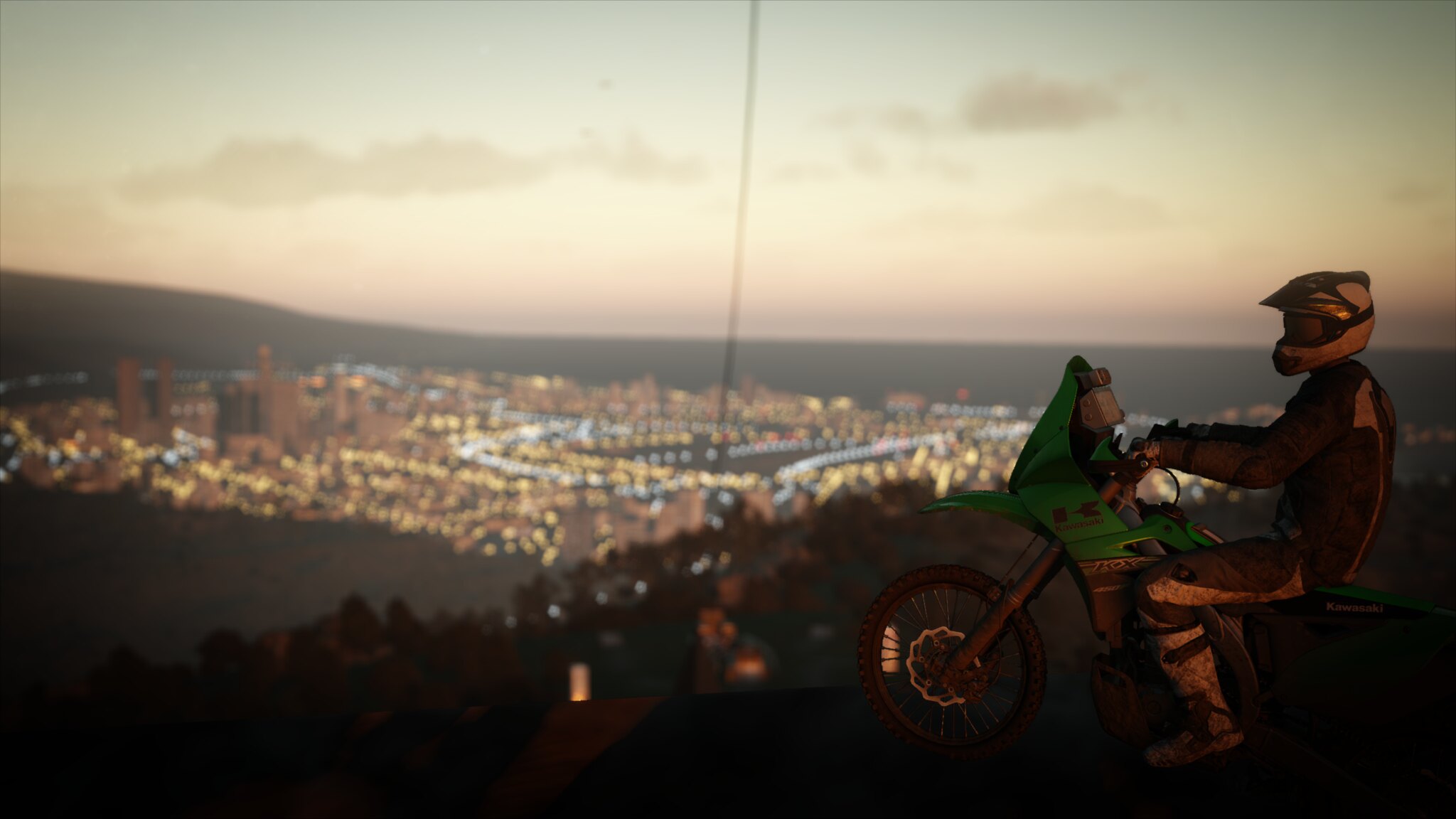A motorcyclist, clad in a gray biker suit with white stripes and wearing a white helmet, sits on his green dirt bike at the edge of a cliff. The city sprawls out below in the distance, its lights twinkling against the evening sky. To the left, majestic skyscrapers rise up, forming a stunning urban skyline. The sun's last rays bathe the scene in an orange glow, casting a warm light on the motorcyclist, who is positioned to the right of the photo. At the bottom center, the silhouette of the hill's tip where he is perched is visible, highlighting the precarious edge. Far below, the tops of houses and a tree-lined area descend further down the hillside, adding depth to the landscape. The motorcyclist, poised at this breathtaking vantage point, epitomizes the thrill and solitude of the adventure.